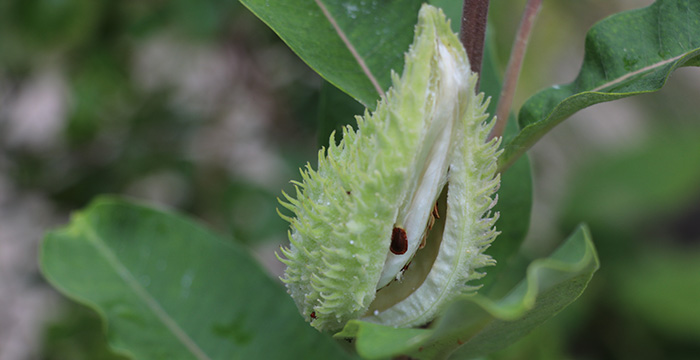This close-up photograph captures a unique pod of an unidentified plant, starting to split open. The pod is pale green and fully cloaked in tiny green, spike-like structures. Its thick, white interior flesh is exposed, revealing brown seeds nestled within. Surrounding the pod, sturdy green leaves and a robust brown stem are visible, providing a stark contrast against the muted, grey overcast backdrop that blurs into indistinct ground and foliage. The overall image evokes a sense of organic complexity, captured in a moment of natural transformation.